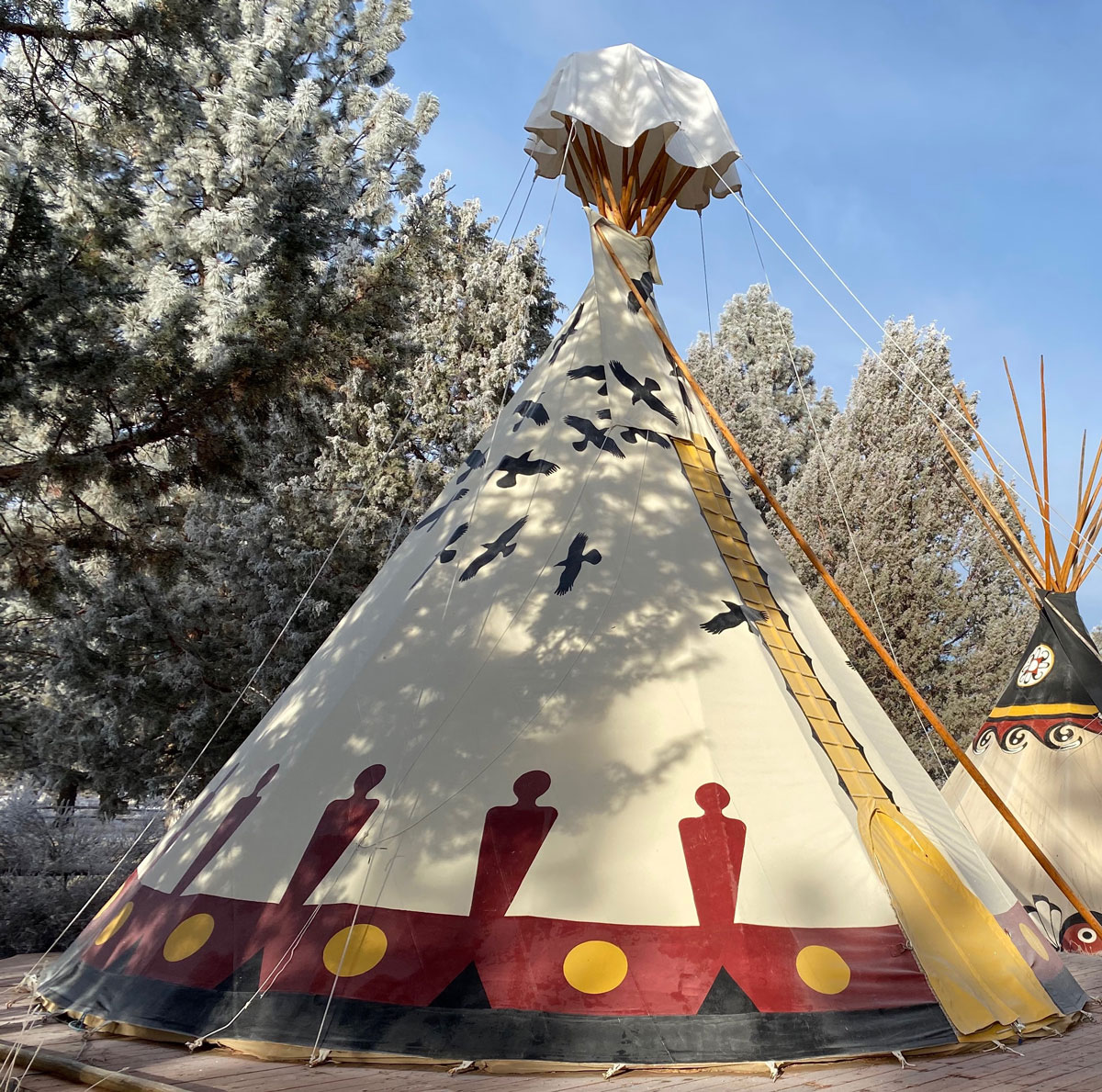The image showcases a picturesque scene featuring two Native American teepees set against a backdrop of snow-covered evergreen trees and a clear blue sky. The teepee in the foreground is predominantly beige with intricate, traditional designs. It features a red and black striped base with small yellow circles evenly spaced within the red stripe. Red, armless human silhouettes are also painted along this base. Above, black birds are silhouetted against the beige fabric, and the right side of the teepee showcases a yellow stripe extending upwards, culminating in an arched yellow flap that appears to serve as a door.

The structure of the teepee is supported by numerous light brown wooden poles that converge at the top, some protruding above the apex and tethered to the ground by thin white strings. The uppermost part of the teepee is covered by a small tarp held down by these strings, adding a modern touch to the traditional design.

To the right and partially cut off from view, stands a second teepee, similarly beige, with its own red, yellow, and black decorations. Unlike the first, this teepee's wooden poles at the top are unshielded by a tarp. Both teepees rest on a wooden platform that blends with the light brown hues of the poles. The serene setting and detailed artistry on the teepees create a harmonious blend of cultural heritage and natural beauty.